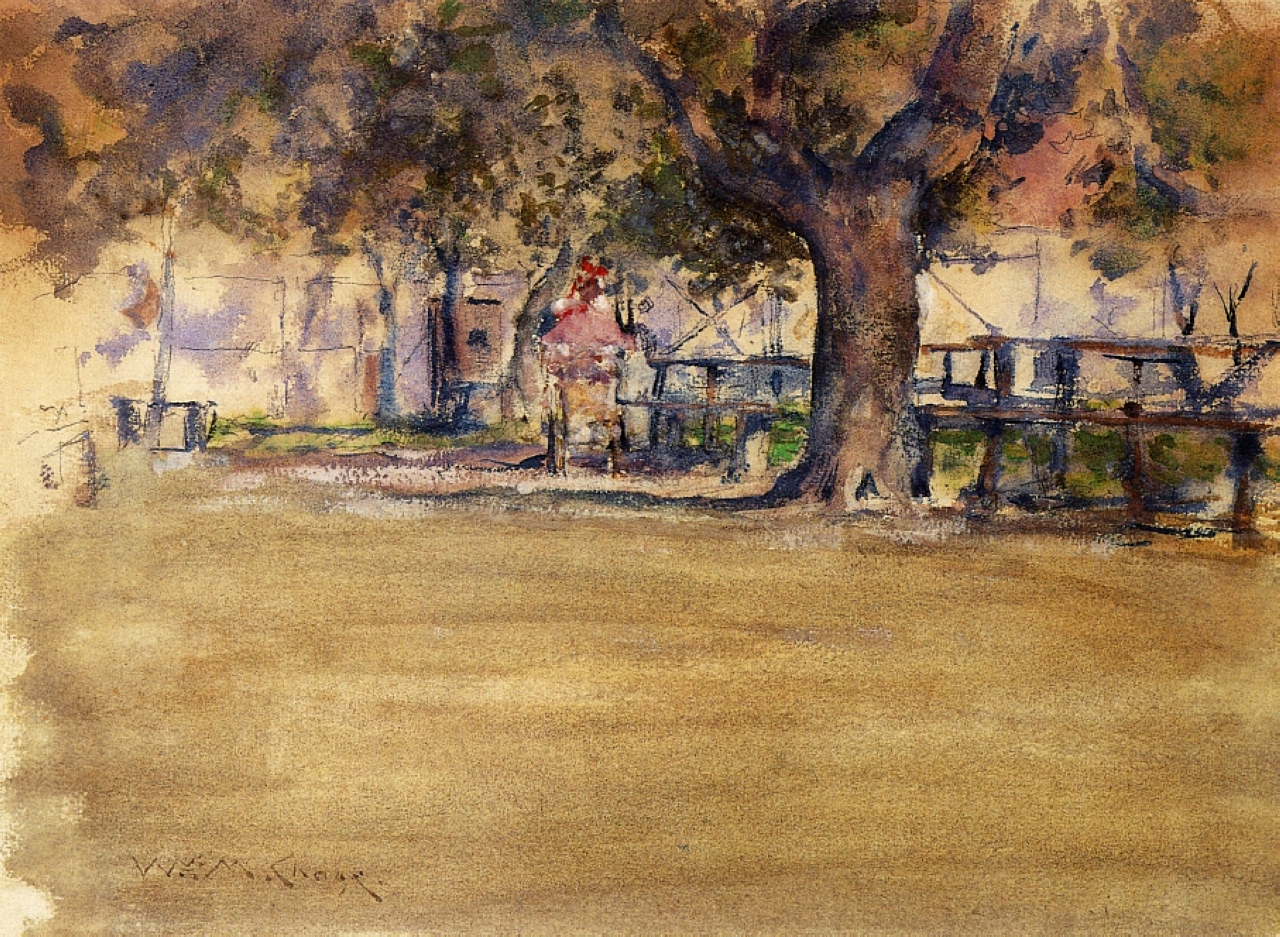The painting illustrates a park-like setting, possibly in the evening, dominated by a large, thick-trunked tree in the foreground. The tree, with its wide, curving branches, is adorned with a mix of green leaves and some areas of moss, creating a dense canopy that slightly hangs low. Surrounding this primary tree are other trees with leaves in varying shades of green, brown, and gold. 

The lower half of the scene features expanses of light brown, dirt-covered ground, interspersed with patches of lighter areas suggesting worn grass. In the background, to the right and left, hazy outlines of buildings are visible, sketched in thin, bold lines, with elements such as a red and gold door standing out. Shadows from the trees play across the white walls of these buildings, adding depth.

Near the tree, there’s a hint of a walkway, along with indistinct forms that might be fences or tables. Additionally, there’s an ambiguous figure in the center, possibly a person, showing pink with red and brown hues. Overall, the composition is reminiscent of a schoolyard or a park, evoking a tranquil, shaded atmosphere.